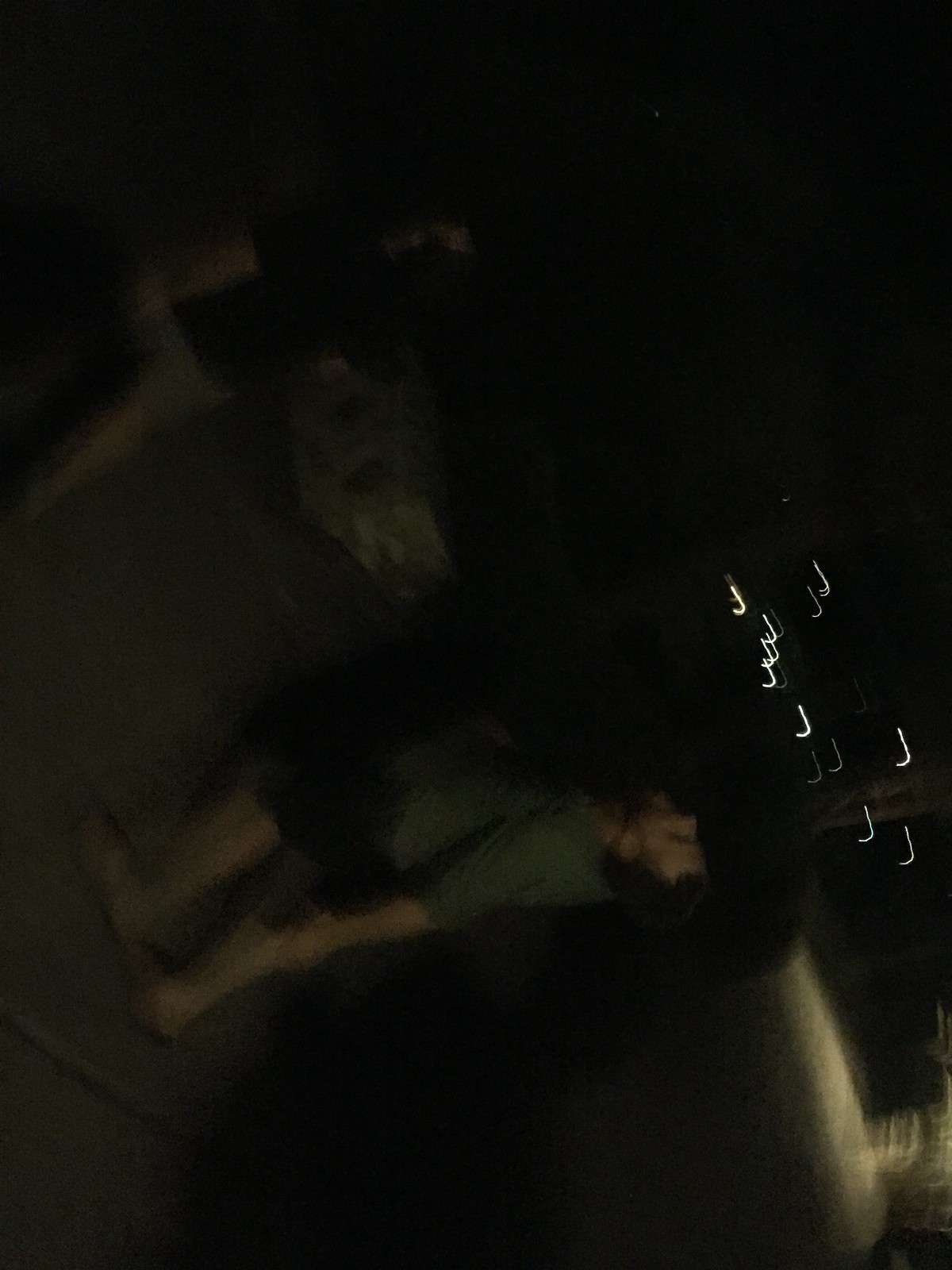A grainy nighttime photograph prominently features an indistinct white male figure, who appears to be leaning backward and looking toward the right-center of the image. He is barefoot and dressed in an elbow-length, round-neck t-shirt and dark-colored shorts. The background is predominantly black, with the exception of some blurred lights in the center-right, which form the shape of the letter 'J' due to camera motion. The figure's feet are positioned at the lower left-hand side, suggesting he was originally standing on the left side of the frame. The entire image seems to be rotated 90 degrees, adding to its overall disorienting nature.